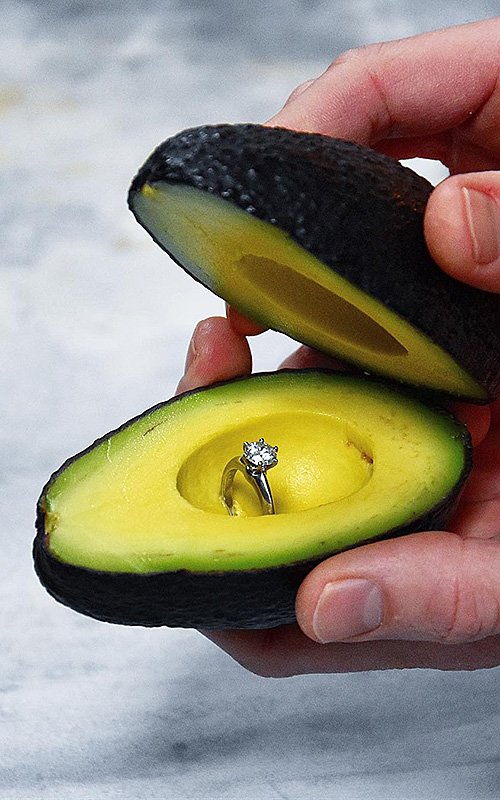This image is a tall, narrow digital photograph featuring an avocado that has been cut in half, with the pit smoothly removed and replaced by a diamond engagement ring. The avocado halves are held open by a man's clean, though unmanicured, hands, which are emerging from the right side of the photograph—his right hand holding the top half and his left holding the bottom. The avocado's vibrant green flesh contrasts with the yellow-green inner flesh, and the whole scene is set against a gray marble surface. This clever composition emulates the look of a traditional jewelry box, using the avocado to creatively present the engagement ring.